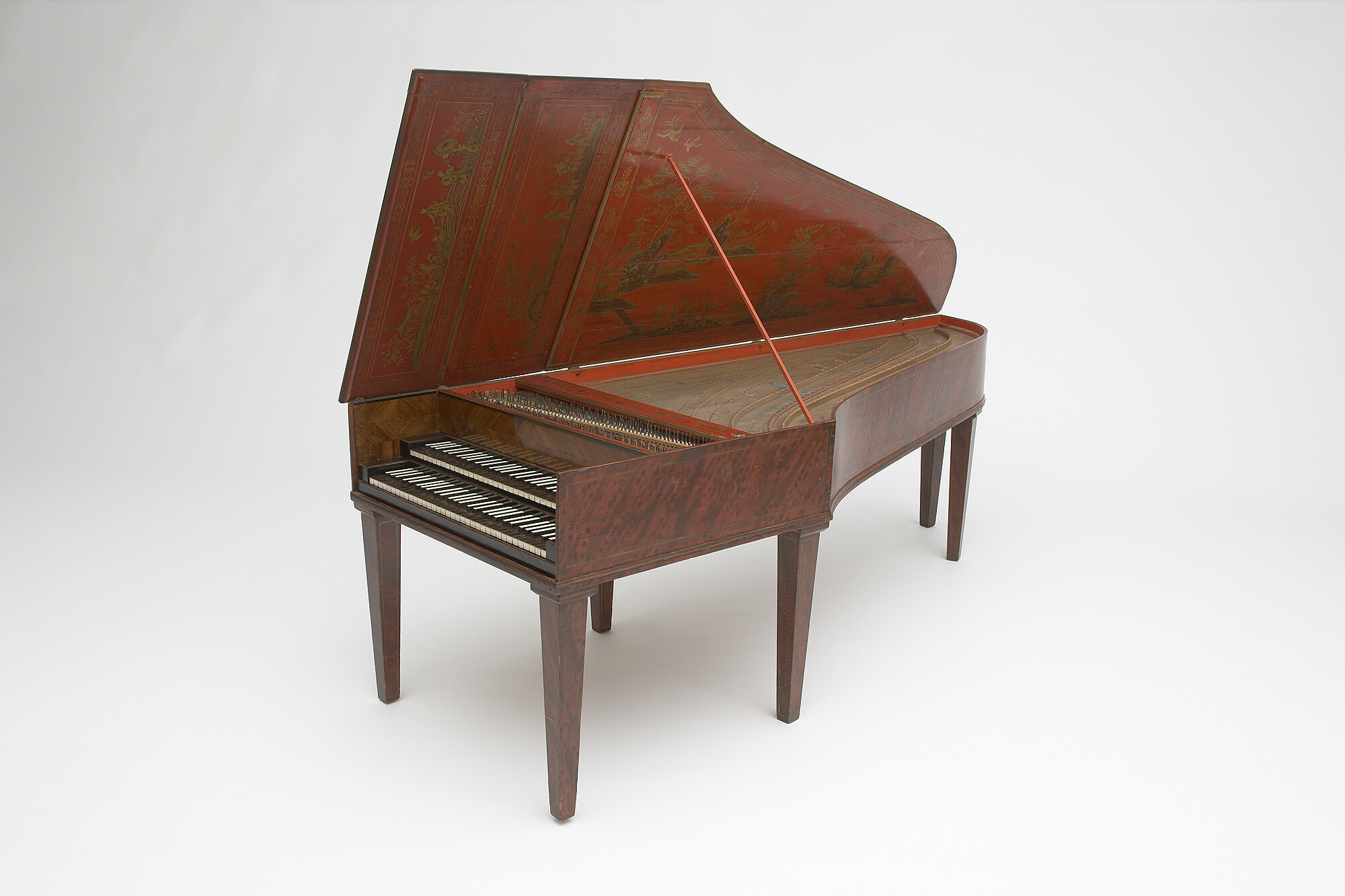The photograph showcases an antique harpsichord, prominently featured against a light gray studio backdrop. The harpsichord is a rich reddish-brown hue, adorned with intricate oriental designs in black and gold on its underside, visible as the lid is propped open. The unique instrument, with its double-deck keyboard layout, displays two rows of keys—black keys positioned below white ones—adding a distinctive character. The structure, supported by six visible legs with possibly a seventh hidden from view, combines a wide and square front with a tapered, angled back. The harpsichord’s body, with its red and black spotted wooden exterior, is a stunning centerpiece in this detailed, indoor photograph.